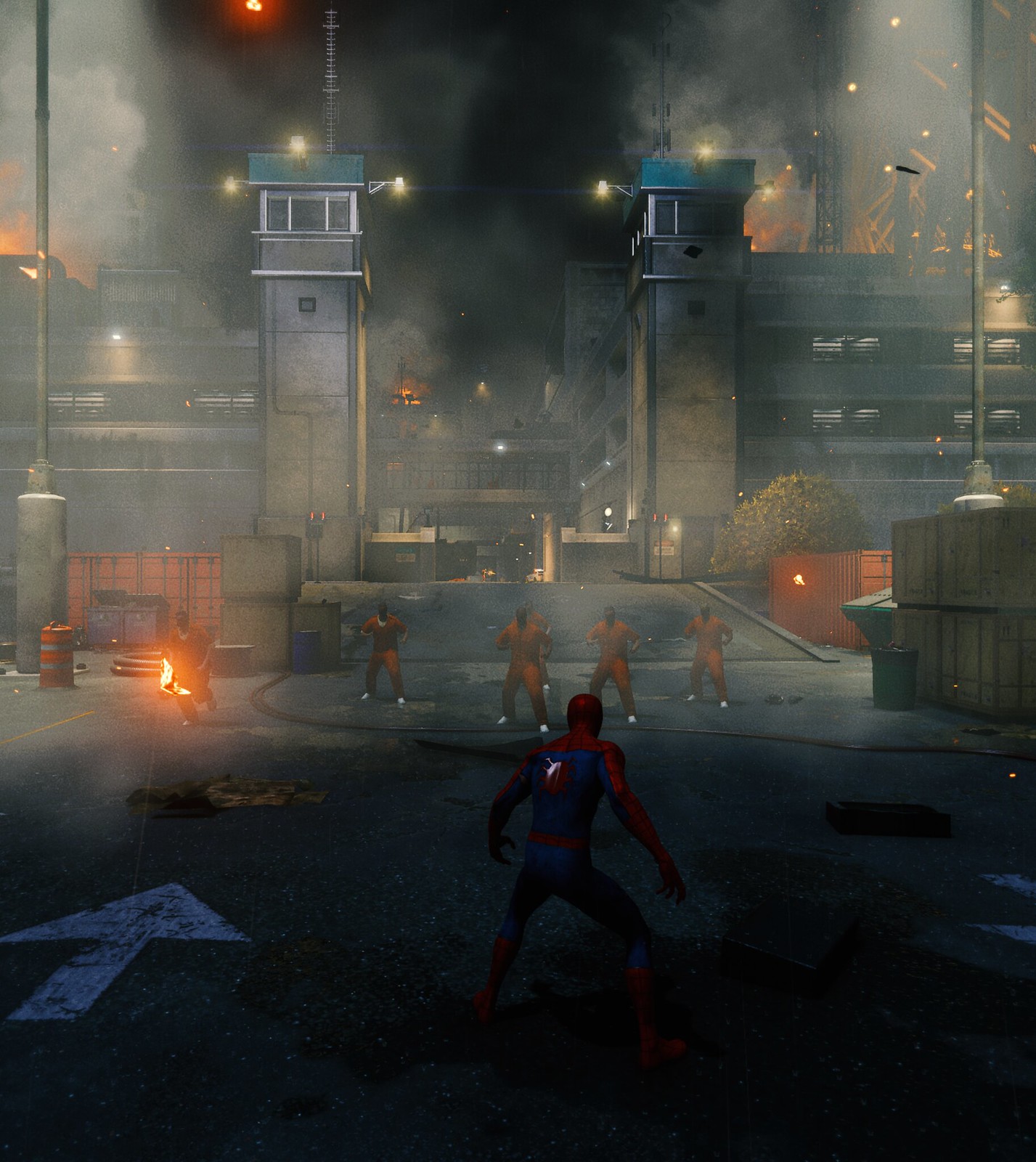In this rectangular, cartoon-like scene that appears to be taken from a video game, we are immersed in a dark, ominous cityscape. At the bottom center of the image, the iconic superhero Spider-Man is visible from the back, easily identifiable by his distinctive red and blue costume. He stands poised, seemingly ready to engage, as he faces six adversaries. These six individuals, aligned horizontally in a fighter's stance, are all clad in orange outfits reminiscent of prison jumpsuits, suggesting they may be escaped convicts. In the background looms a large building that could be a jail, accentuated by the pervasive glow or fire emanating from its roof, casting an eerie light over the nighttime setting. No text interrupts this tense moment; the scene is solely conveyed through its dramatic imagery.